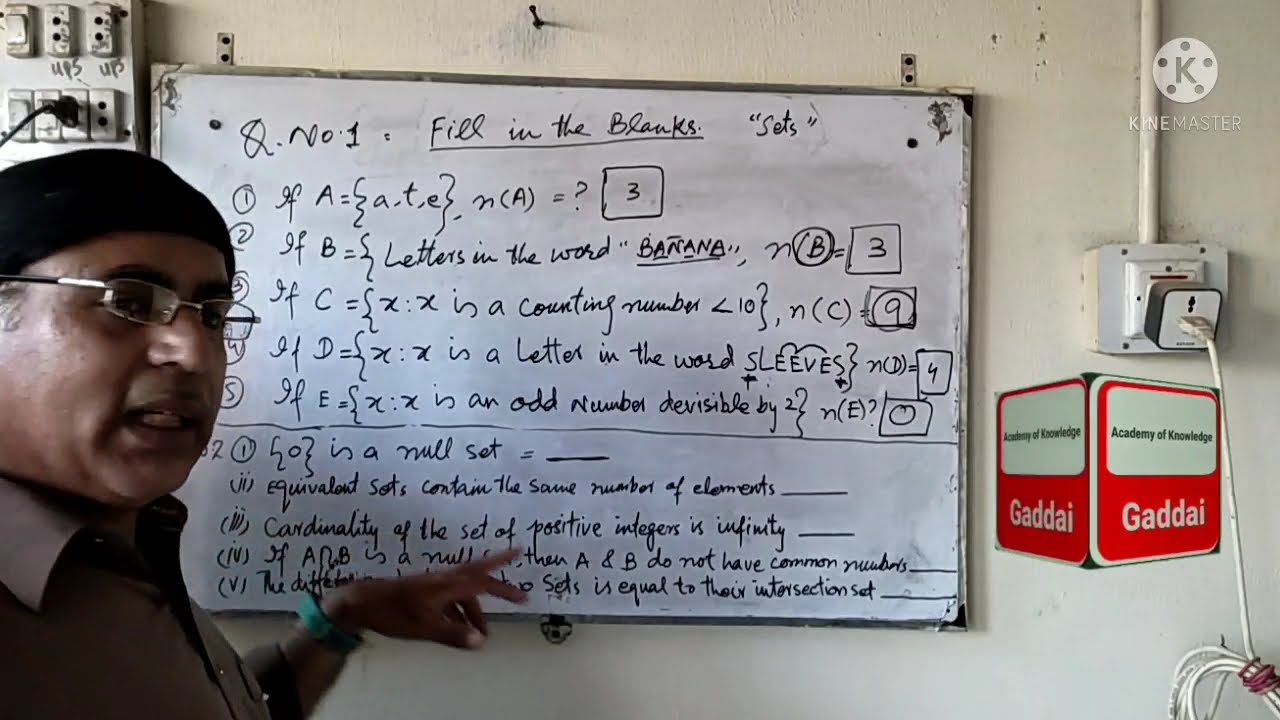The image depicts a man of Indian descent, likely a teacher, standing in front of an old whiteboard mounted on an off-white painted wall. He is wearing metal-framed glasses, a black knit tassel cap, and a brown collared shirt. He has a green wristwatch on his left wrist, which he uses to point at the handwritten text on the whiteboard. The text includes a series of formulas and questions under the heading "fill in the blanks." To the right of the whiteboard, an electrical outlet with visible wiring is present, along with a device plugged into it. There is also a sticker on the wall that reads "Academy of Knowledge GADAI" twice, with a reflective effect. A circular logo with the letter "K" at the top and the words "Khan Master" below it is also visible near the whiteboard. This classroom scene combines detailed elements such as the man's attire, the text on the whiteboard, and various items on the wall, providing a comprehensive view of the educational setting.